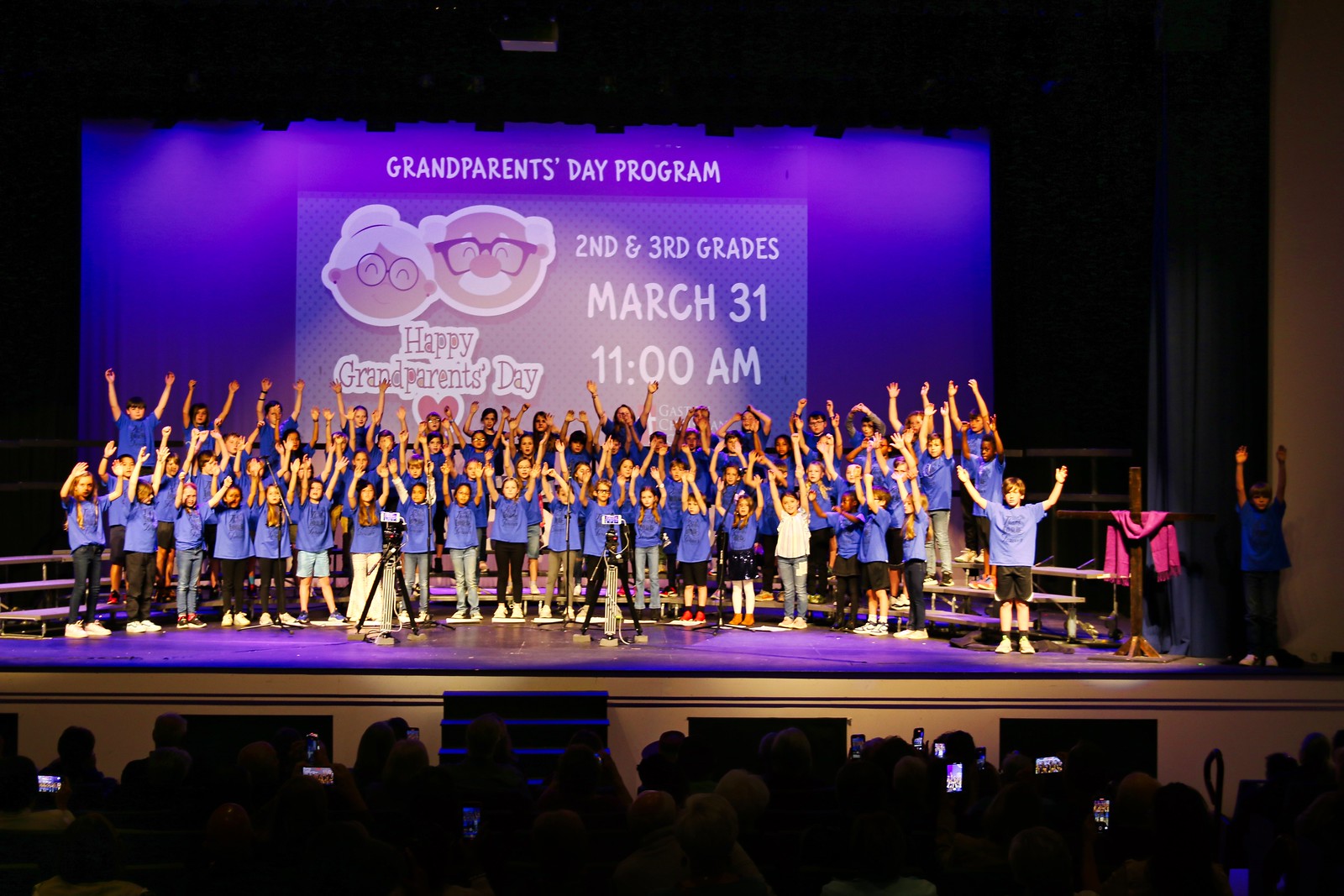The photograph captures an indoor school assembly celebrating Grandparents' Day. The rectangular image, viewed from the audience, shows the backs of heads in the foreground and darkly lit auditorium. The stage, illuminated and primarily colored in purple with beige accents near the top, features three rows of children, approximately 20 per row, all wearing purple t-shirts and raising their hands in celebration. Behind them, a large electronic screen displays "Grandparents Day Program, Second and Third Grades, March 31st, 11 a.m." in white text against a purple background. The screen also shows two cartoon drawings of a smiling elderly man and woman, adorned with the message "Happy Grandparents Day." To the right-hand side of the stage, a wooden cross draped with a red scarf is visible, along with a little boy separated from the main group of children.